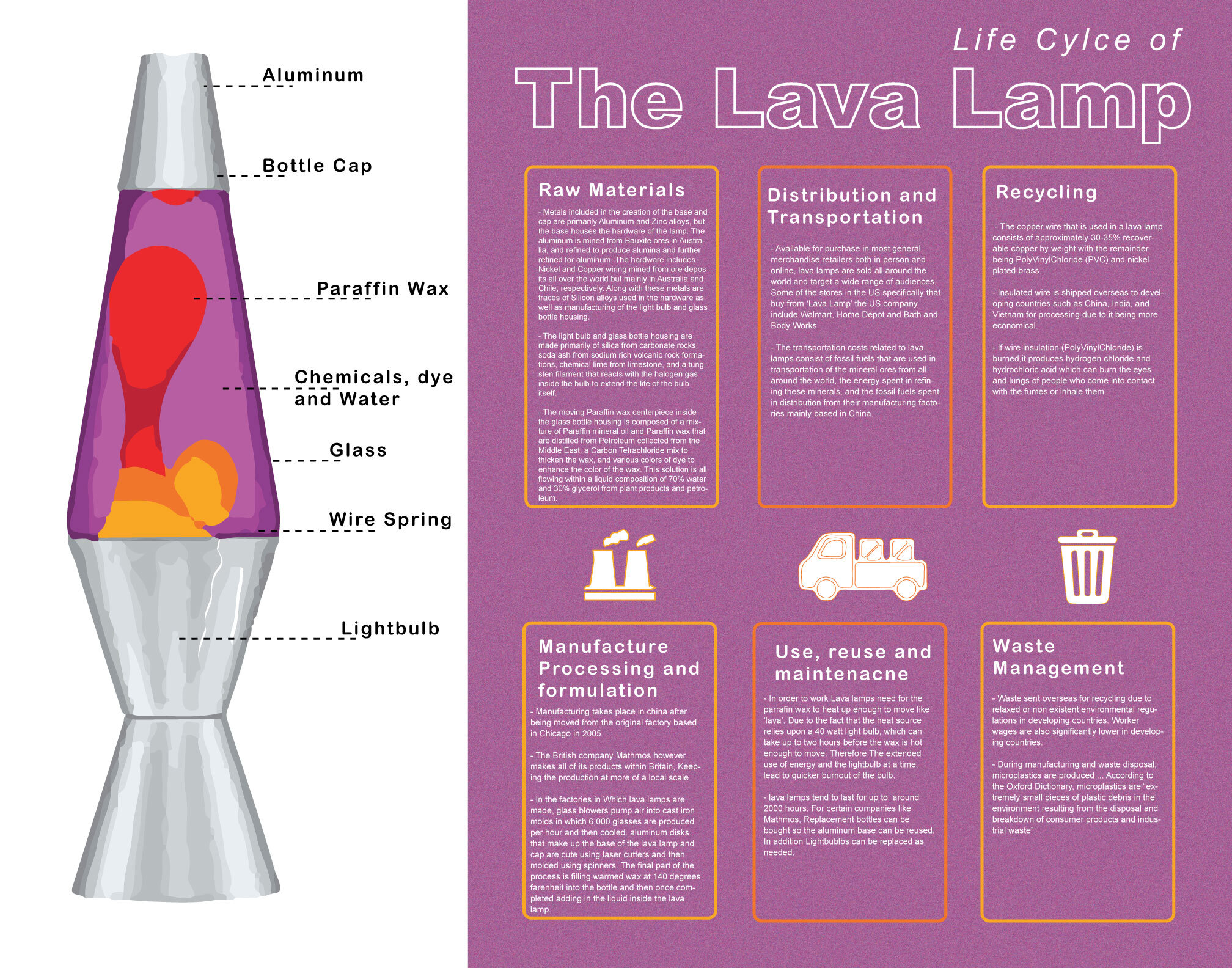This image is an informational diagram highlighting the life cycle and anatomy of a lava lamp. Dominantly purple in color, the diagram is divided into a left and right section. On the left, a detailed cartoon drawing of a standard silver-topped and silver-based lava lamp is presented. Arrows and dotted lines point to various components, labeling them as follows: aluminum bottle cap (top), paraffin wax (lava mixture), chemicals, dye, and water (liquid inside), glass (outer structure), wire spring (base connection), and light bulb (heating element). 

To the right of the lava lamp diagram, a large purple info box features the heading "Life Cycle of the Lava Lamp" in a white outline font. Under this heading, six orange rectangles are arranged in two rows of three, each representing a distinct phase of the lava lamp's life cycle. The phases are listed as: 

1. Raw Materials
2. Distribution and Transportation
3. Recycling
4. Manufacture, Processing, and Formulation
5. Use, Reuse, and Maintenance
6. Waste Management

Beneath each rectangle, small white icons depict related images, such as a factory, truck, and trash can. Each box also contains detailed text explaining the respective phases, though the text is too small to read clearly in the image. The overall design is visually cohesive, emphasizing the flow and lifecycle of a lava lamp through detailed annotations and structured segments.